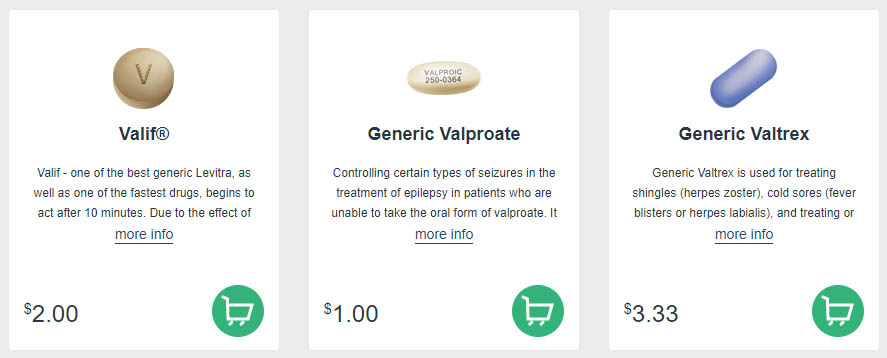This detailed description captures the visual and textual elements on a small cropped screenshot from a pharmaceutical app or website.

---

The screenshot showcases a section of a pharmaceutical app or website with a light blue background, where three different pills are listed within white boxes. Each listing features details about the medication, including names, images, descriptions, and pricing.

1. **Valif**:
    - **Position**: Leftmost box
    - **Title**: "Valif" in black letters
    - **Pill Image**: A round, brown pill with the letter "V" at its center
    - **Price**: $2 displayed at the bottom left
    - **Purchase Option**: Green circle with a shopping cart icon at the bottom right
    - **Additional Info**: Description text below the title

2. **Valproate**:
    - **Position**: Center box
    - **Title**: "Valproate" along with a lot number
    - **Pill Image**: Displayed at the top
    - **Description**: Labeled as "generic Valproate"
    - **Price**: $1 displayed at the bottom left
    - **Purchase Option**: Shopping cart icon at the bottom right

3. **Generic Valtrex**:
    - **Position**: Rightmost box
    - **Title**: "Generic Valtrex"
    - **Pill Image**: A round, purple capsule
    - **Price**: $3.33 displayed at the bottom left
    - **Purchase Option**: Shopping cart icon at the bottom right

The structured layout within the white boxes contrasts against the light blue background of the website, organizing and highlighting the essential information clearly.